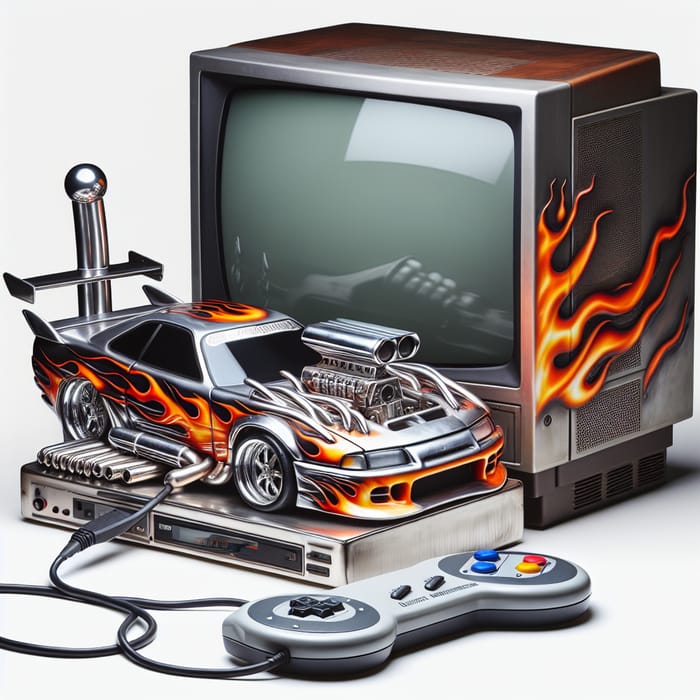The image depicts an artistic rendering of a retro Nintendo game console and a small, old-fashioned box TV. The game console is exceptionally slim and silver-colored, with a black cable leading to a distinctive controller, which features blue, yellow, and red buttons on the right side, two controls in the middle, and a square control on the left. The TV, likely from the 90s and reminiscent of those equipped with VHS players, has a brown top with silver metal lining and a blank gray screen. Both the console and the TV are embellished with fiery red and orange flame decals, lending a dynamic and retro aesthetic. Atop the console sits a silver sports car model, characterized by its large, exposed engine protruding through the hood, numerous pipes, a prominent spoiler, and flame designs on the top, sides, and front. This incorporation of flames across the car, console, and TV adds a cohesive and vibrant theme to the scene.